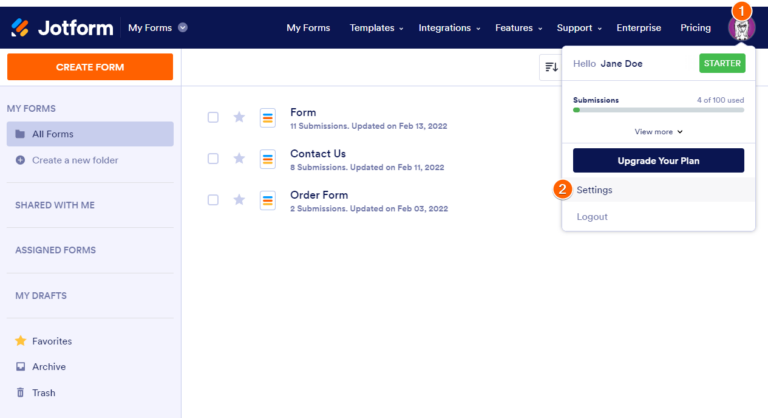The image is a detailed snapshot of the JotForm web page. On the left side, there's a colorful logo followed by the word "JotForm" in white, stylized, folded font. To its right, "My Forms" is displayed in white font along with a dropdown menu. Extending from slightly left of center to the right, in white font, are the menu items: "My Forms," "Templates," "Integrations," "Features," and "Support," each accompanied by a dropdown menu, followed by "Enterprise" and "Pricing." A small purple icon with a white interior and an orange circle featuring the number "1" in white, bordered by white, is visible.

On the far left, inside a light purple area, there's an orange button labeled "Create Form" in white letters. Below it, the sidebar displays options like "My Forms," "All Forms," and "Create a New Folder," each with corresponding icons. Further down, separated by light lines, are sections titled "Shared with Me," "Assigned Forms," "My Drafts," "Favorites" (with a yellow star icon), "Archive," and "Trash."

The central area of the page lists forms with their corresponding details: "Form" with 11 submissions updated on February 13, 2022; "Contact Us" with 8 submissions updated on February 11, 2022; and "Order Form" with 2 submissions updated on February 3, 2022. Each form entry includes icons, unfilled stars, and empty square checkboxes.

On the right, a pop-up greets "Jane Doe" (bolded). It displays "Starter" in green with white font and continues with a submission count, "4 of 100 used," followed by a "View More" link. Below it, a navy blue button invites the user to "Upgrade Your Plan" in white lettering, and additional options including "Settings" (flagged with a number 2 in an orange circle) and "Log Out."